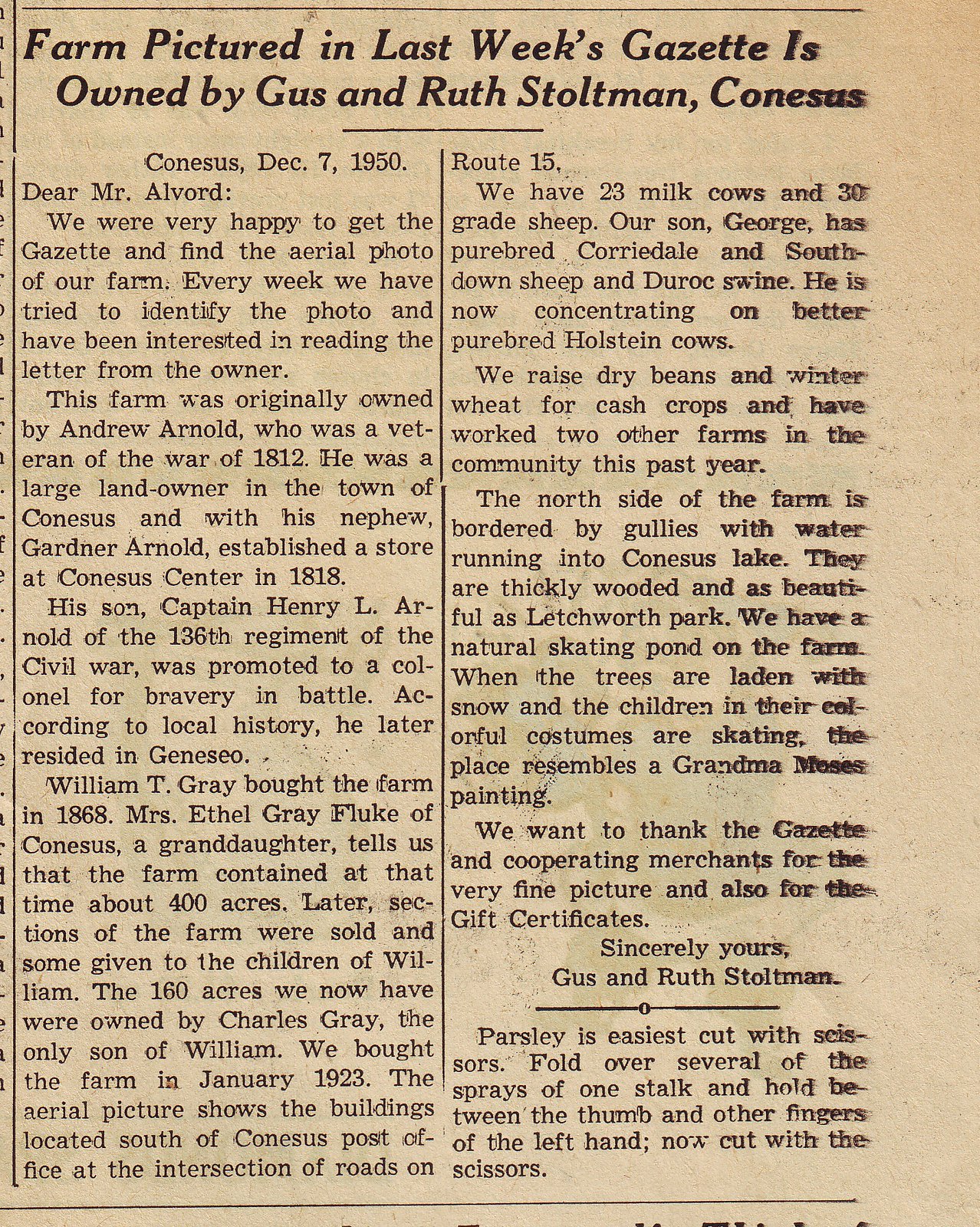The image captures a yellowed newspaper clipping from December 7, 1950. Prominently at the top in bold text, it reads: "Farm Pictured in Last Week’s Gazette is Owned by Gus and Ruth Stoltman, Kinesis." The article, marred slightly on the right side by ink blurring due to age, is a letter to Mr. Alvord. Gus and Ruth Stoltman express their delight in seeing the aerial photo of their farm in the Gazette. They recount their farm’s rich history, noting that it was originally owned by Andrew Arnold, a War of 1812 veteran, who also established a store in Kinesis Center in 1818 with his nephew, Gardner Arnold. Further historical milestones include Captain Henry L. Arnold of the 136th Regiment in the Civil War being promoted to colonel for bravery, and William T. Gray acquiring the farm in 1868, which at the time spanned around 400 acres. Many sections were later distributed among William's children. The Stoltman’s current 160-acre holding was owned by Charles Gray before they purchased it in January 1923. The letter details their farming activities—maintaining 23 milk cows, 30 grade sheep, and raising Corydale and Southdown sheep and Durock swine. They also cultivate dry beans and winter wheat and work two additional farms. Featured in the aerial photo are the farm's buildings located south of Kinesis Post Office at the intersection of Route 15. The farm's picturesque north side, with thick woods and gullies, borders Kinesis Lake, often resembling a Grandma Moses painting during winter with children skating on their natural pond. The Stoltman’s close by thanking the Gazette and local merchants for the aerial picture and gift certificates.